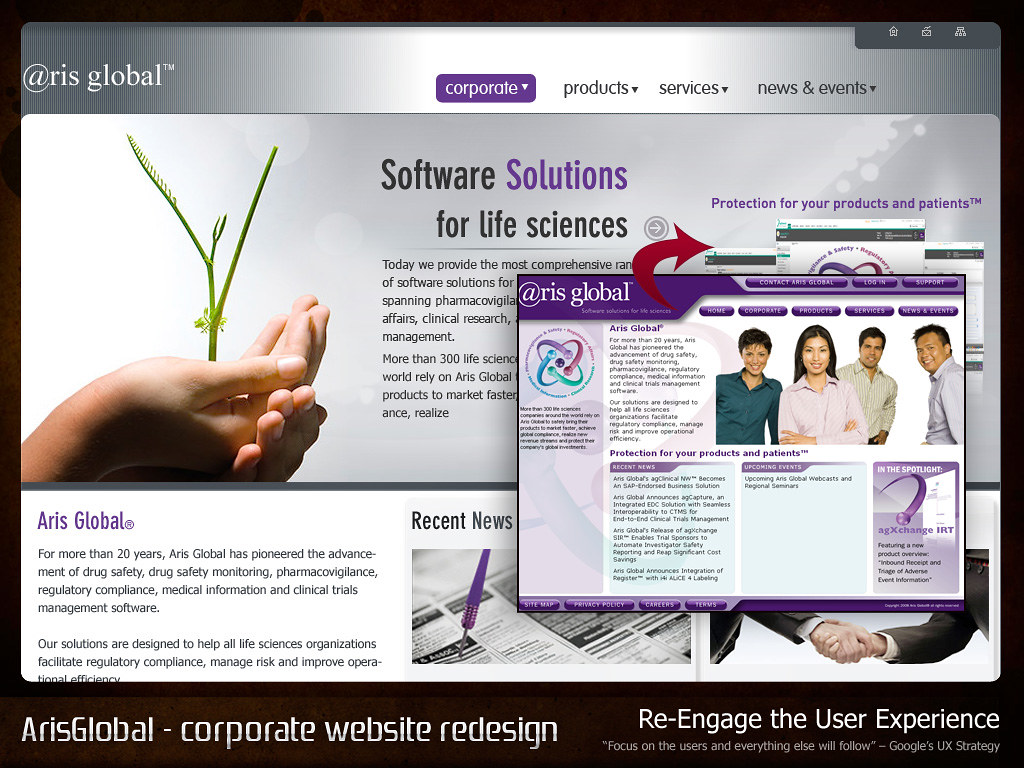The large, square image advertises a software company, likely as part of a website redesign prototype. Encased in a black border, the upper part of the image transitions from dark gray on the left to light gray and white on the right. In the upper-left corner, "@RIS Global" is written in white text. Dominating the top portion is a large rectangular section with a white and gray background, featuring the phrase "Software solutions for life sciences," where "solutions" is highlighted in purple while the rest of the text is black. Below this, two paragraphs of left-aligned text are partially obscured by a pop-up square box showing "@RIS Global" again. This overlay contains a photo of two women and two men, with more text arranged in various columns.

The image evokes a web page's layout, complete with a top menu bar listing "Corporate Products," "Services," "News," and "Events." The background of the webpage shifts from silver to white, and then back to silver. On the left of the main section, there is a picture of two hands holding a green sprout, adjacent to the phrase "Software solutions for life sciences." 

In the lower white-background section of the image, "ARIS Global" appears in purple, accompanied by text that reads: "For more than 20 years, ARIS Global has pioneered the advancement of drug safety, drug safety monitoring, pharmacovigilance, regulatory compliance, medical information, and clinical trials management software." This area also features another paragraph that's partly cut off by the bottom black border, which states "ARIS Global Corporate Website Redesign" and "Re-engage the user experience." The overall design suggests this is an ad or a presentation showcasing a proposed redesign of the ARIS Global corporate website.